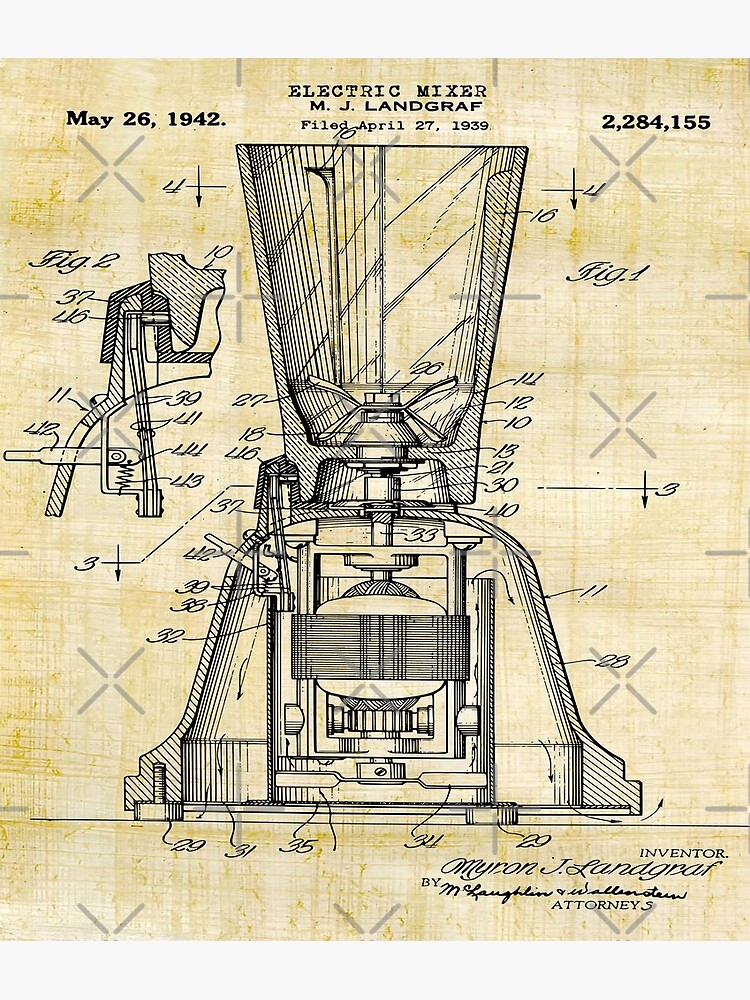This is a detailed engineering diagram of an electric mixer, identified as patent number 2,284,155, filed by M.J. Langraff on April 27, 1939, with a notation dated May 26, 1942. The stenciled drawing depicts a blender-like device with a glass reservoir at the top, housing blender blades. A complex cross-section of the base reveals the internal motor, complete with multiple numbered labels likely explained in an accompanying document. The diagram, characterized by its intricate and labeled design, showcases a sophisticated motor and mechanical components indicative of pre-World War II American innovation. The entire image features watermark X's and black font annotations detailing patent information and inventor credentials, emphasizing the elaborate and technical nature of this early 20th-century invention.